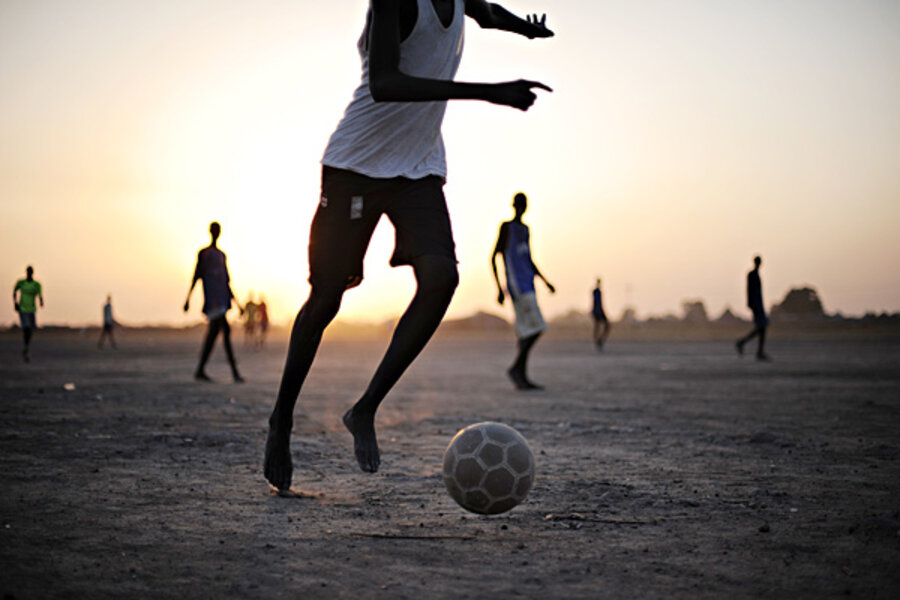The photograph, taken at dusk, captures a dynamic scene of children playing soccer on a sandy or dirt-covered field. The central figure in the foreground, who is barefoot, is mid-action about to kick a soccer ball with gray panels and white seams. The child is dressed in a white tank top and black shorts cut above the knees. Despite the blurred depth of field, other players in the background, some wearing blue or green shirts, are visible and appear to be enough to form a team, making up nine figures in total. The image, exhibiting professional quality, shows an expansive, open field with minimal obstacles and low-level trees in the distant background, along with indistinct structures or hills. The setting sun casts a warm glow, emphasizing the evening atmosphere.